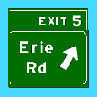In this image, there is an extremely small depiction of a traffic sign typically found on highways. The sign features a light blue square-shaped background that serves as its outer frame. At the bottom of the sign, the words "Erie Rd" (an abbreviation for Erie Road) are displayed in white text against the light blue backdrop. Adjacent to this text, an arrow points diagonally upward to the right, indicating direction. Above the Erie Road sign, there is a rectangular sign with the white text "Exit 5" positioned on its right side. This rectangular sign is bordered by a thin, dark gray square-shaped line that forms an outer barrier around the sign itself.